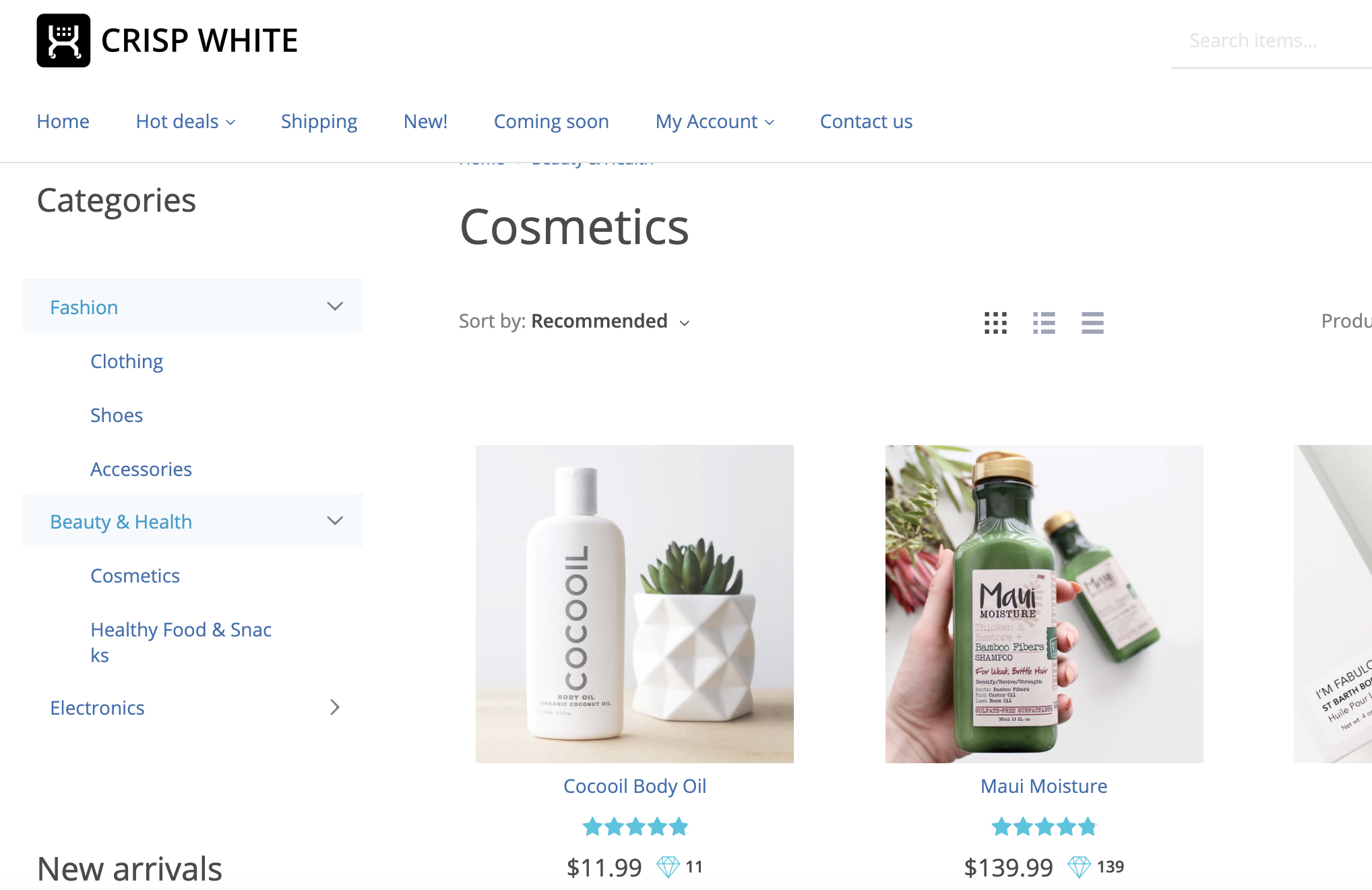At the top of the image, there is a black square with a unique design in the middle, beneath which the words "Crisp White" are written. Below this, a blue menu displays several options: "Home," "Hot Deals," "Shipping," "New," "Coming Soon," "My Account," and "Contact Us." There is also a search bar labeled "Search Items." On the left side, a sidebar lists various categories: "Fashion," "Clothing," "Shoes," "Accessories," "Beauty and Health," "Cosmetics," "Healthy Food and Snacks," "Electronics," and "New Arrivals." On the right side, at the top, there is a large heading that says "Cosmetics," followed by sorting options "Sort by Recommended." Featured prominently below this is an image of a plastic bottle labeled "Cocoa Oil" and a flower pot with aloe or a similar plant growing in it. The product, "Cocoa Oil Body Oil," is rated five stars and priced at $11.99. A blue diamond icon with the number 11 is displayed on the right side of the product description.